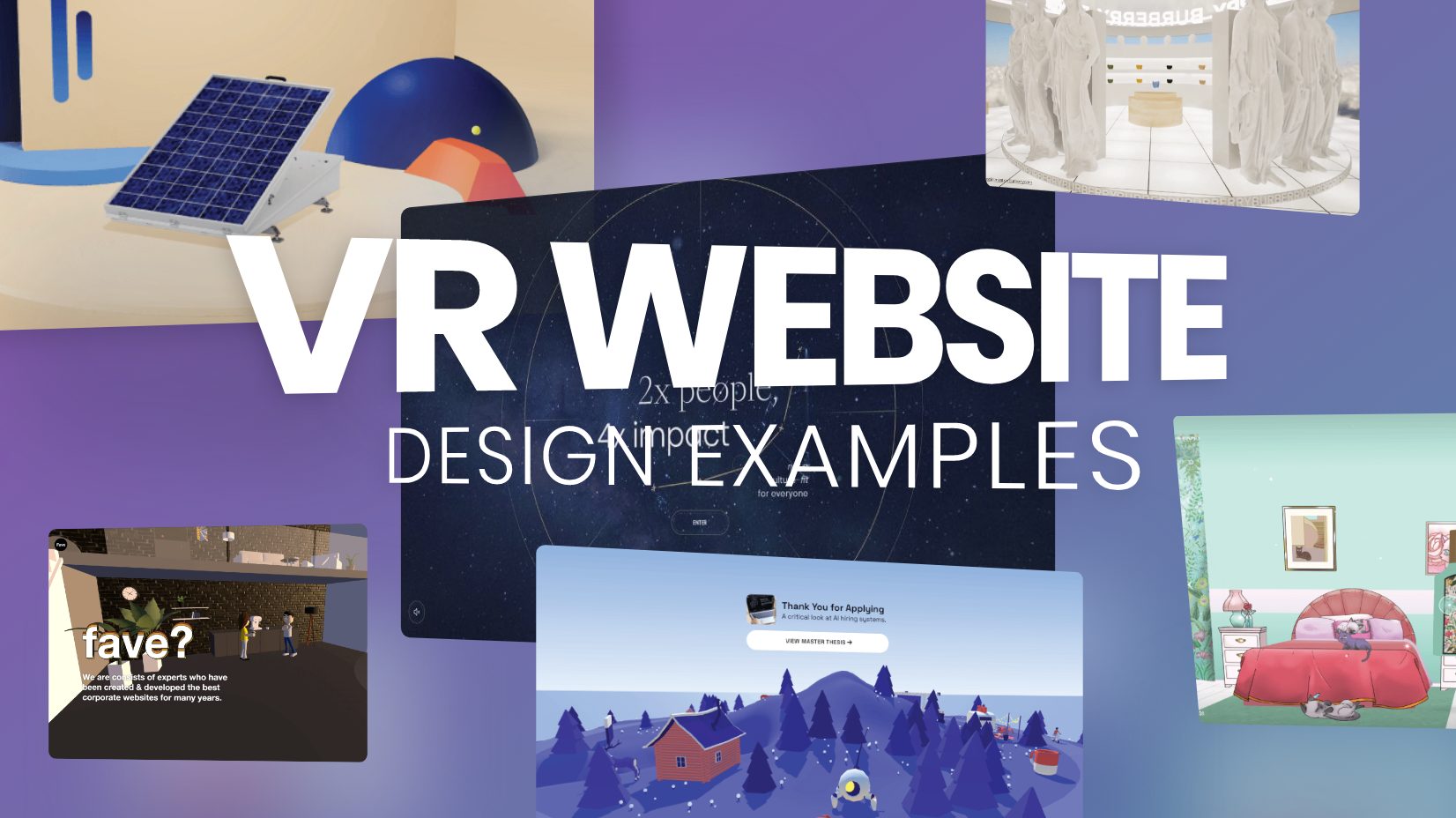The image is a widescreen rectangular graphic featuring the centered title "VR WEBSITE DESIGN EXAMPLES" in bold, bright white, capital letters. The background showcases a gradient transition from purple to blue, particularly noticeable towards the bottom right corner. Surrounding the title are six floating website design examples, with five partially visible. Notable images include a platform in the top right, a bedroom scene in the bottom right, and a solar panel in the top left. The middle display might represent a website's home screen featuring the text "Two times people, four times impact." The setup suggests that this is either an advertisement or a stock photo intended for VR software-related content.